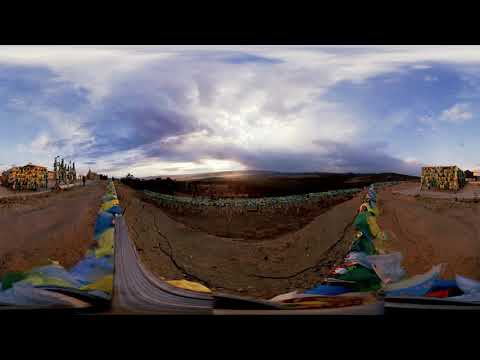The image depicts a dynamic and colorful landscape with an intense sky above. The top half of the image showcases a vibrant sky filled with an array of clouds, suggesting either a sunrise or sunset as the sun peeks out from behind them, casting dramatic light and shadows. Below this dramatic sky, the ground is composed of sandy and dirt-covered terrain, forming a central dip or trough resembling a u-shape, filled with a mix of vivid colors including green, yellow, blue, red, grays, and whites, suggesting a distorted perspective or artistic effect. On either side of this trough, dirt pathways or ramps traverse the terrain, implying the image might be viewed from the standpoint of someone driving through or riding over these features, such as on a motorcycle. The left and right sides of the image feature indistinct structures; the one on the left appears next to a road lined with buildings and some poles in front of it, while the structure on the right side remains square and unclear. Both sides cradle the central trough that dips and then rises again on each edge. In the foreground, the multicolored paths extend from left to right and down the sides of the trough, adding to the dynamic and surreal quality of the scene.